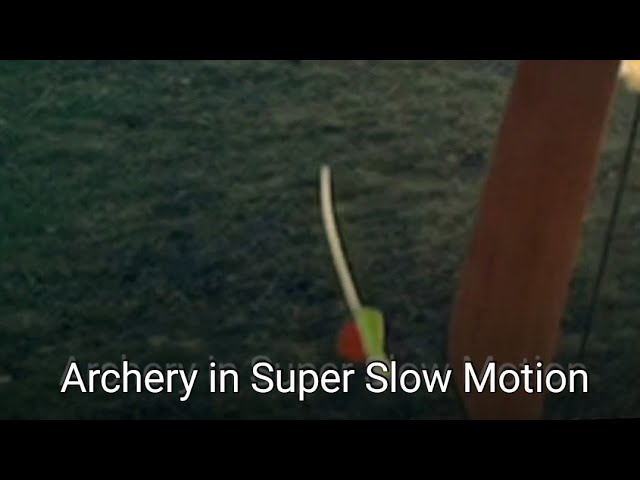The image appears to be a thumbnail from a paused YouTube video titled "Archery in Super Slow Motion," as indicated by the white text at the bottom of the screen. The scene is in letterbox format with black bars at the top and bottom, giving it a cinematic feel. The background shows green grass under bright daylight, with sunlight visible in the top right corner. In the foreground, there's a wooden archer's bow with a black string on the right-hand side, and an arrow, partway released, flying towards the left. The arrow is crafted from blonde wood, featuring a white tip and vibrant fletching with red and green feathers. The details emphasize the meticulous craft of archery, captured in stunning slow motion.